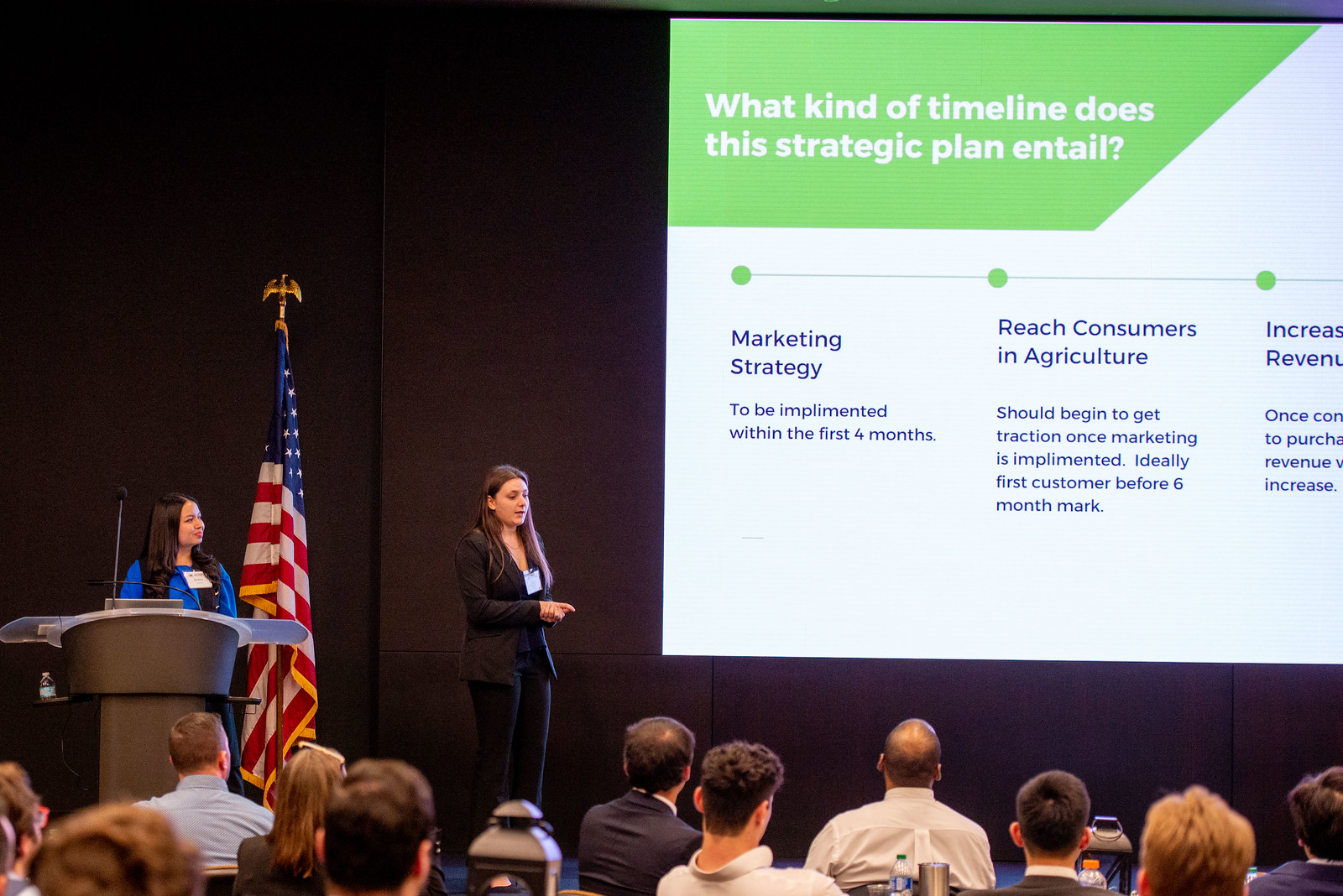This image captures a detailed scene of a conference presentation. The setting is a conference room with a brown back wall and a large screen displaying a PowerPoint slide. The slide, featuring green and white with blue text, reads, "What kind of timeline does this strategic plan entail?" It outlines key points: a marketing strategy to be implemented within the first four months, reaching consumers in agriculture, ideally securing the first customer before the six-month mark, and an incomplete point about increasing revenue. On stage, to the left, there's a podium and behind it an American flag. Two women are present; one wearing a blue jacket stands behind the podium, while the other, dressed in a fitted black pantsuit, engages with the audience. The woman in the black suit has long brown hair and points toward the crowd, capturing the interest of the seated audience members, who appear attentive and professionally dressed.